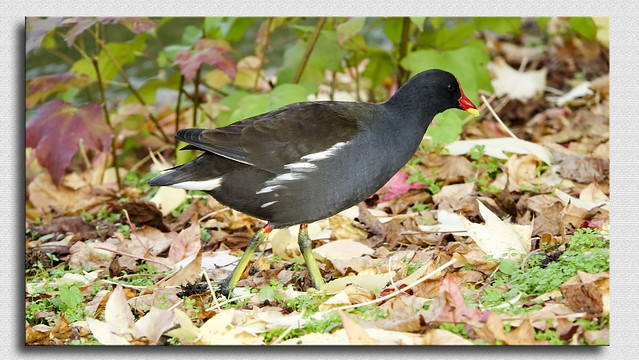The image is a close-up, color photograph taken outdoors, featuring a dark-feathered bird primarily seen from a side angle. The bird's plumage is predominantly black with touches of white just under its wings and at the tail. It has a striking reddish-orange beak with a yellow tip and beady black eyes that blend into its dark face. A distinctive red band can be seen at the top of its legs, which are otherwise yellowish and appear tall and wiry, though its feet are obscured by the brown, dead leaves it walks amongst. The ground is scattered with these dead leaves, interspersed with small green plants resembling four-leaf clovers, and taller plants with brown stems and large, flat green leaves, some of which are dark purple or brown. The bird is moving toward the right side of the frame, seemingly marching through its leafy environment.